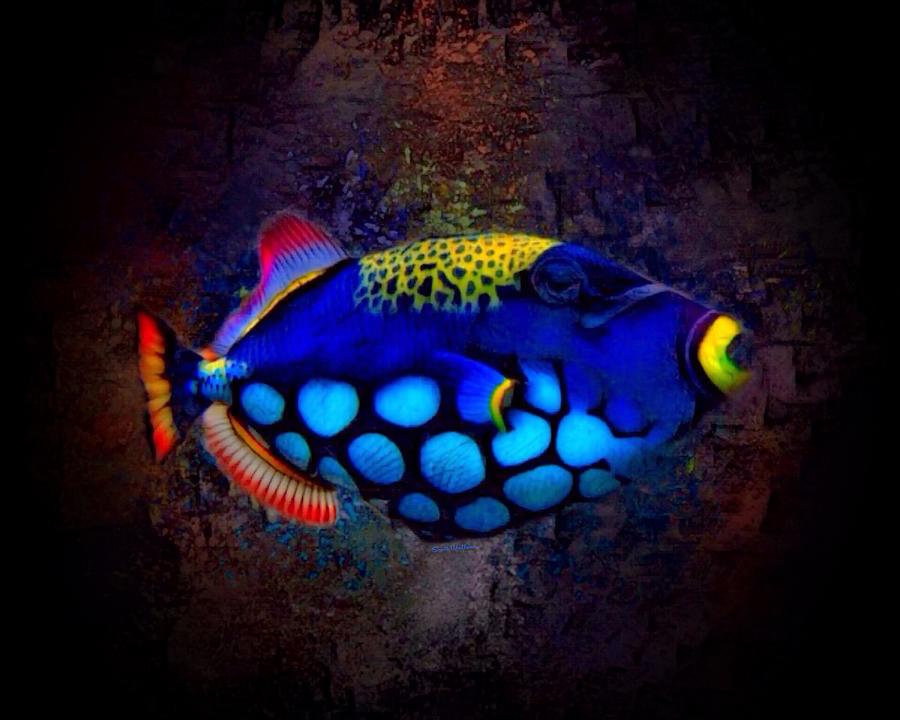The image depicts an intricately detailed piece of artwork featuring a vibrant tropical fish against a contrasting black and iridescent background. The backdrop includes a brown stone wall illuminated with shades of light green, dark green, light blue, and dark blue light. The corners of the image fade into black, drawing the viewer’s focus to the colorful fish in the center, which is oriented facing right.

The fish itself is predominantly blue with a vibrant yellow marking on its top, dotted with black, and a striking yellow eye. Its belly is adorned with light blue spots outlined in black. The fish has an array of vivid fins; the top fin features shades of red and blue, while the bottom fin, near the tail, is a mix of white and red. Its tail starts as black at the base and transitions into a blend of red and yellow at the end. The detailed artwork, possibly painted, captures the fish’s intricate and mesmerizing colors, infusing a sense of depth and movement.